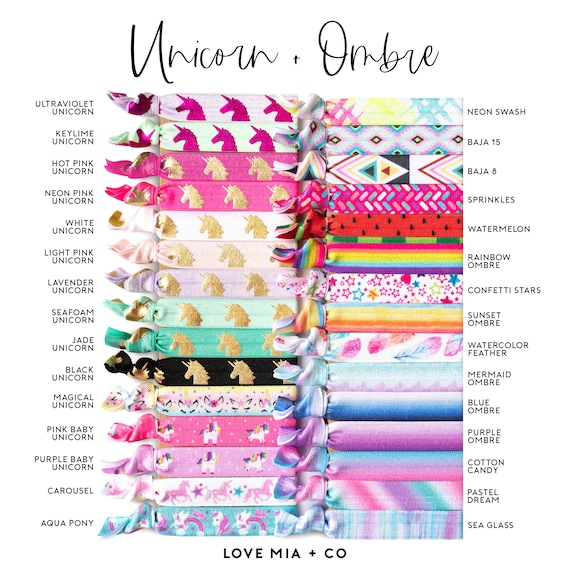In the image, a vibrant and diverse collection of fabric swatches, marketed as "Unicorn + Ombre," are displayed. The assortment showcases both unicorn-themed and ombre-patterned materials, each meticulously labeled. The unicorn fabrics on the left include ultraviolet unicorn, key lime unicorn, hot pink unicorn, neon pink unicorn, white unicorn, light pink unicorn, lavender unicorn, seafoam unicorn, jade unicorn, black unicorn, magical unicorn, pink baby unicorn, purple baby unicorn, and carousel aqua pony. The ombre fabrics on the right feature neon swash, Baja 15, Baja 8, sprinkles, watermelon, rainbow ombre, confetti star, sunset ombre, watercolor feather, mermaid ombre, blue ombre, purple ombre, cotton candy, pastel dream, and sea glass. These swatches, with their bright, fun, and girlish colors ranging from vivid pinks to subtle greens and blues, suggest applicability for crafting and quilting. The top of the image is branded with "Unicorn + Ombre," and the bottom includes the label "Love Mia and Co," hinting at the company behind these whimsical designs, likely targeted towards a market favoring colorful and imaginative fabric options for creative projects.